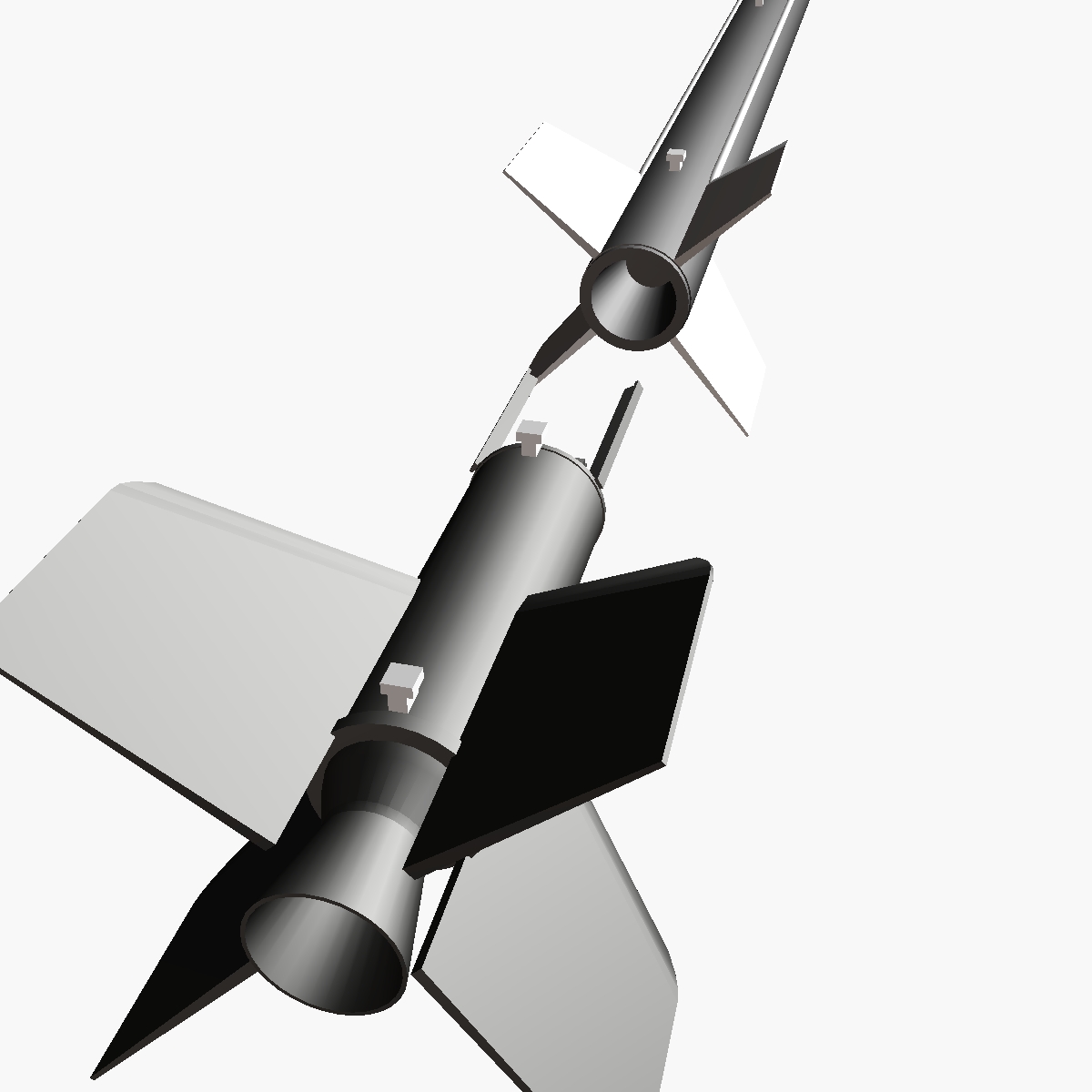The image is a computer-drawn graphic of a rocket, depicted in portrait layout with a clear white background. The rocket is shown in two separate stages, aligned diagonally from the upper right to the bottom left corner of the frame. Each stage features four stabilizing fins positioned at the 0, 90, 180, and 270-degree marks. The fins are mostly gray, although some appear black, likely due to shadowing effects.

The main body of the rocket is cylindrical, while the base of each stage flares outward in a cone shape where propulsion would occur. Both stages include white T-shaped objects, positioned towards the bottom and the top on the lower stage and around the middle on the upper stage. The exact function of these objects is unclear. Additionally, at the top of the lower stage, two beams extend outward, suggesting connection points with the upper stage, which appears designed to connect seamlessly. 

The entire image has a minimalist style with no additional context or text, leaving the scale of the rocket ambiguous.